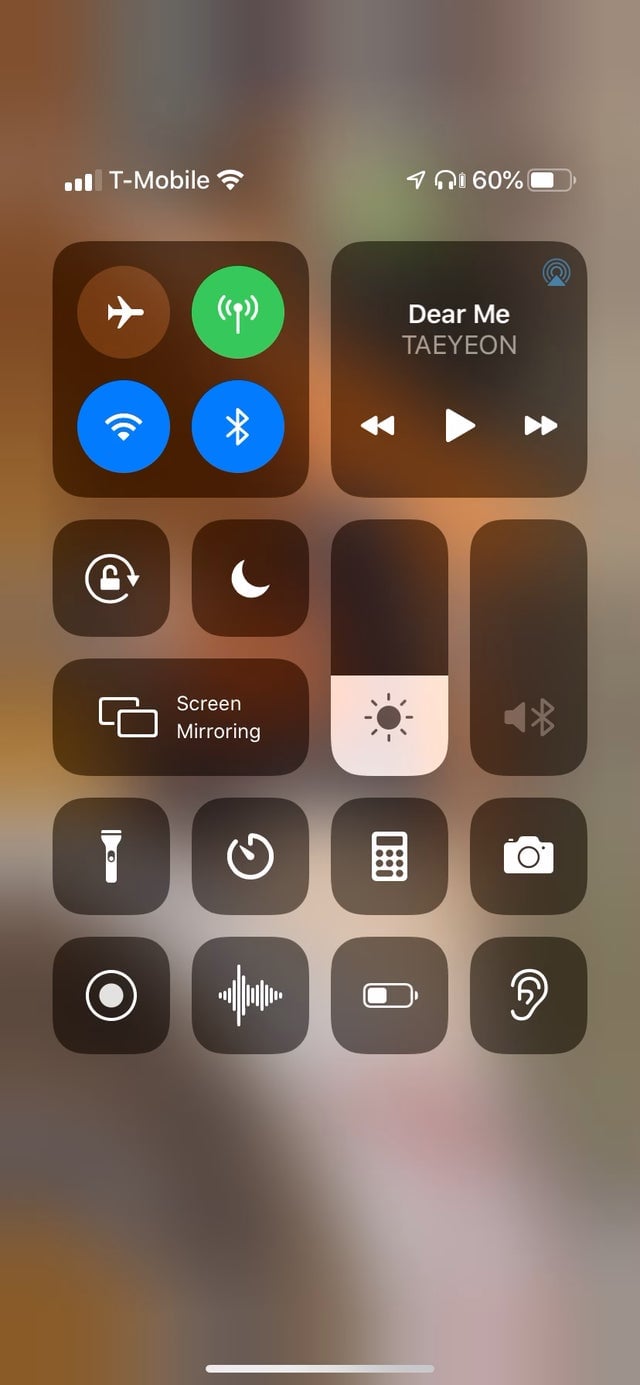This screenshot from a T-Mobile phone captures the pull-down menu of an iPhone. The background is a blurred image, rendering it unidentifiable. The menu items are displayed within darker, cubed sections that stand out against the backdrop.

At the very top, the status bar indicates the network provider, T-Mobile, with cellular service bars to the left and Wi-Fi signal bars to the right. The upper right corner shows a white battery symbol indicating a 60% charge, alongside icons for connected headphones and a navigation arrow.

The pull-down menu is divided into two primary sections. The upper section contains multiple circular icons: an airplane mode icon within a circle, a green circle featuring the Bluetooth symbol, a blue circle for Wi-Fi, and a Do Not Disturb moon icon. Below these, there's a music player widget displaying "Dear Me - Taeyeon," complete with a play button and skip forward/backward controls.

The lower section of the menu includes various essential controls and icons: a lock symbol in a circle for orientation lock, a screen mirroring icon, an adjustable brightness slider, separate Bluetooth control, a flashlight icon, a calculator, a camera icon, a volume slider, and the battery icon.

This detailed configuration offers comprehensive control and quick access to essential iPhone functions, all neatly arranged within the pull-down menu.